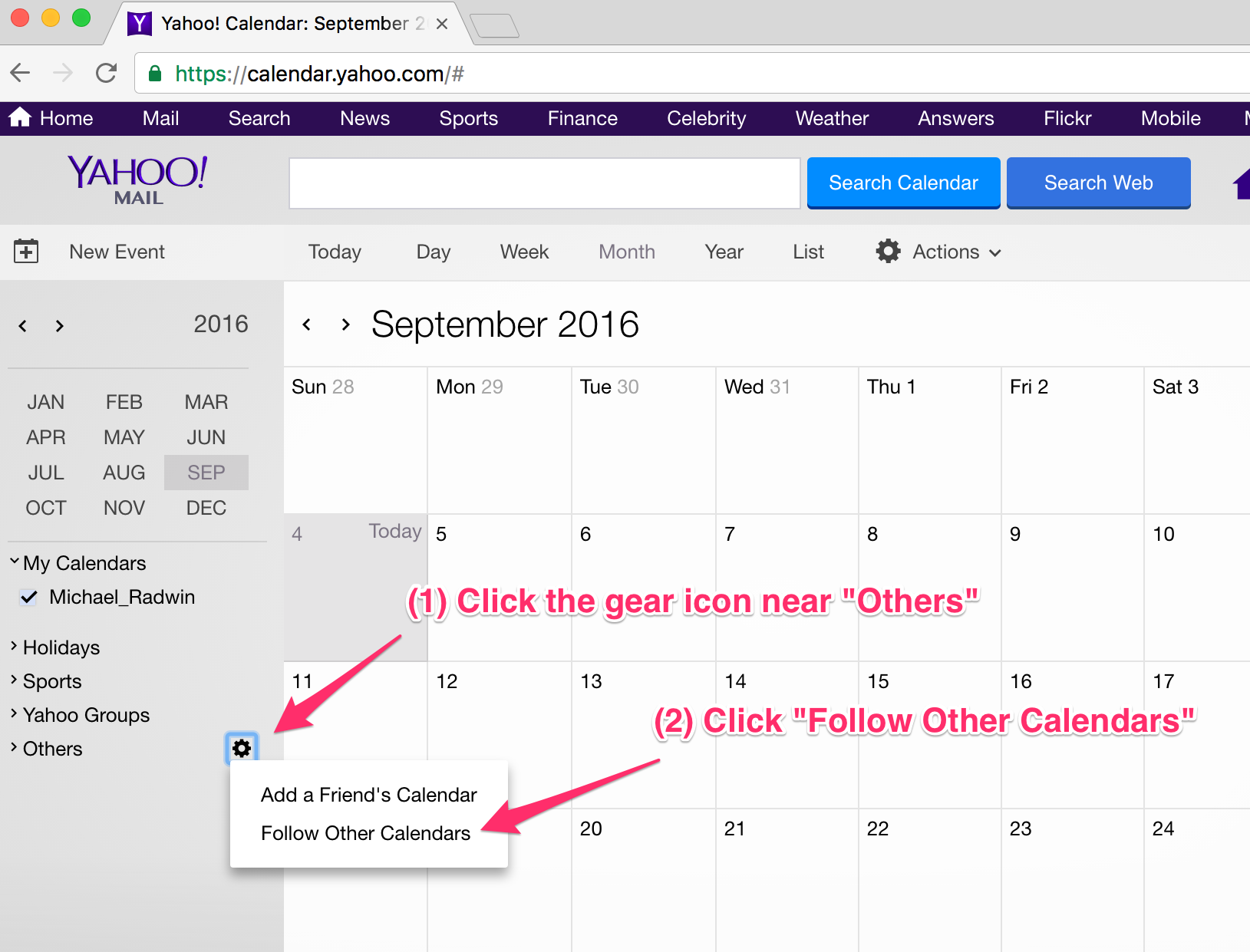The image depicts the Yahoo Calendar interface within a web browser. The browser features a red, green, and orange circle in the top left corner, typical of a macOS window. The browser's address bar displays "calendar.yahoo.com," indicating the URL. Just below the address bar, there is a toolbar with a back button, a refresh button, and a search box with two buttons labeled "Search Calendar" and "Search Web."

The main calendar display shows the month of September 2016 with the first day falling on a Thursday. On the left-hand side, there is a sidebar containing various options and tools. At the bottom of this sidebar, there's a section labeled "Others," which includes a gear icon highlighted by a pink arrow with a "1" in parentheses. A text box emerging from this gear icon states options such as "Add a friend's calendar" and "Follow other calendars." Another pink arrow, labeled "2" in parentheses, points to the "Follow other calendars" option, guiding users to click it.